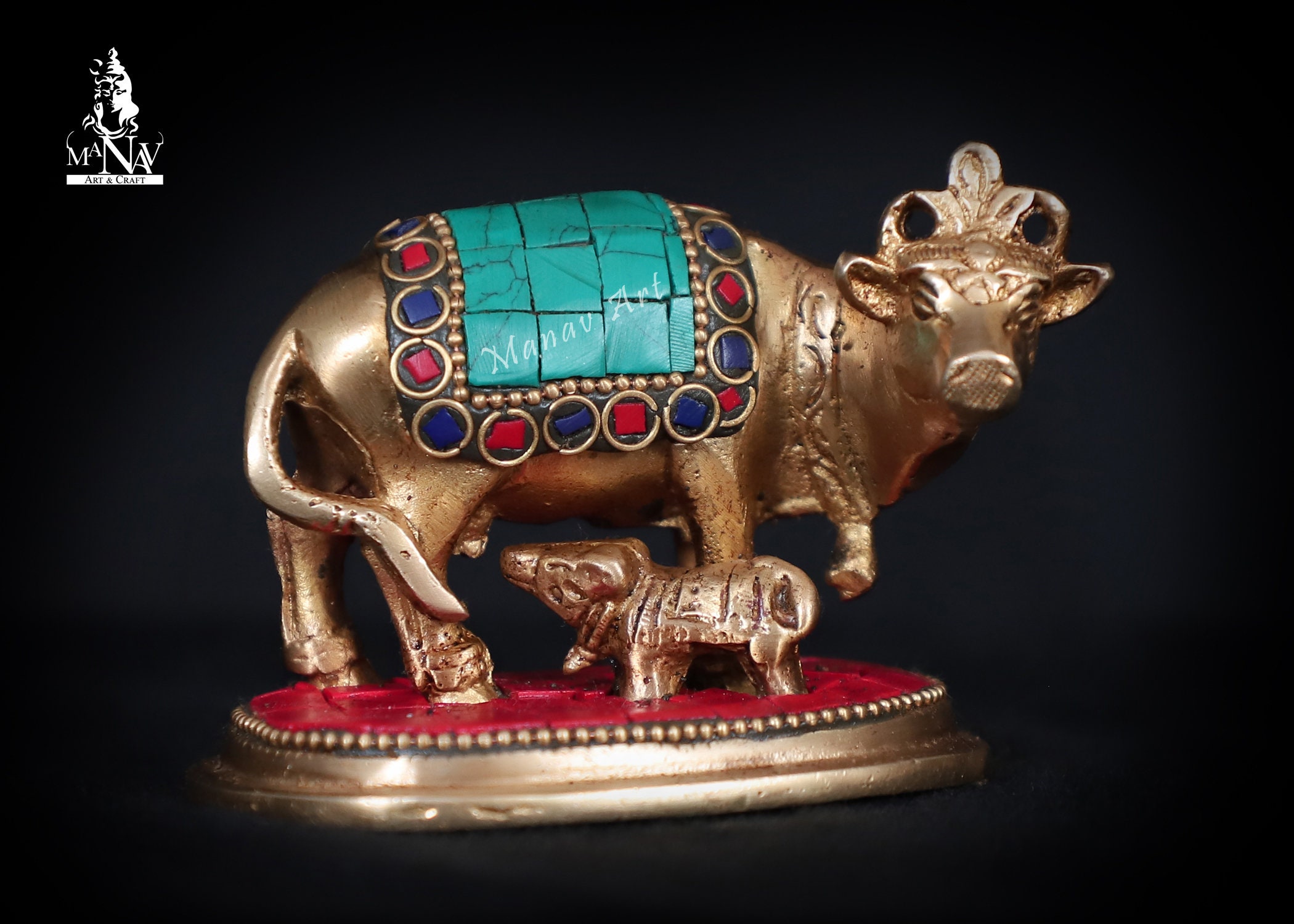The image depicts a meticulously crafted figurine set against a black background. The centerpiece of the artwork is a golden cow adorned with a crown on its head. Drape over the cow's back is a richly designed blanket embellished with gemstones, featuring a turquoise center surrounded by blue and red jewels in an intricate pattern. Below the cow, a golden calf is positioned as if preparing to nurse from its mother. Both the cow and calf stand on an elevated red oval base with gold accents, suggestive of a ruby-like material. Visible blemishes on the craftwork hint at the handmade nature of this artistic piece. In the upper right corner of the photograph, the words "M-A-N-A-V, MANAV, Art and Craft" are displayed along with an image of a goddess, adding context and significance to the figurine’s cultural and artistic value.